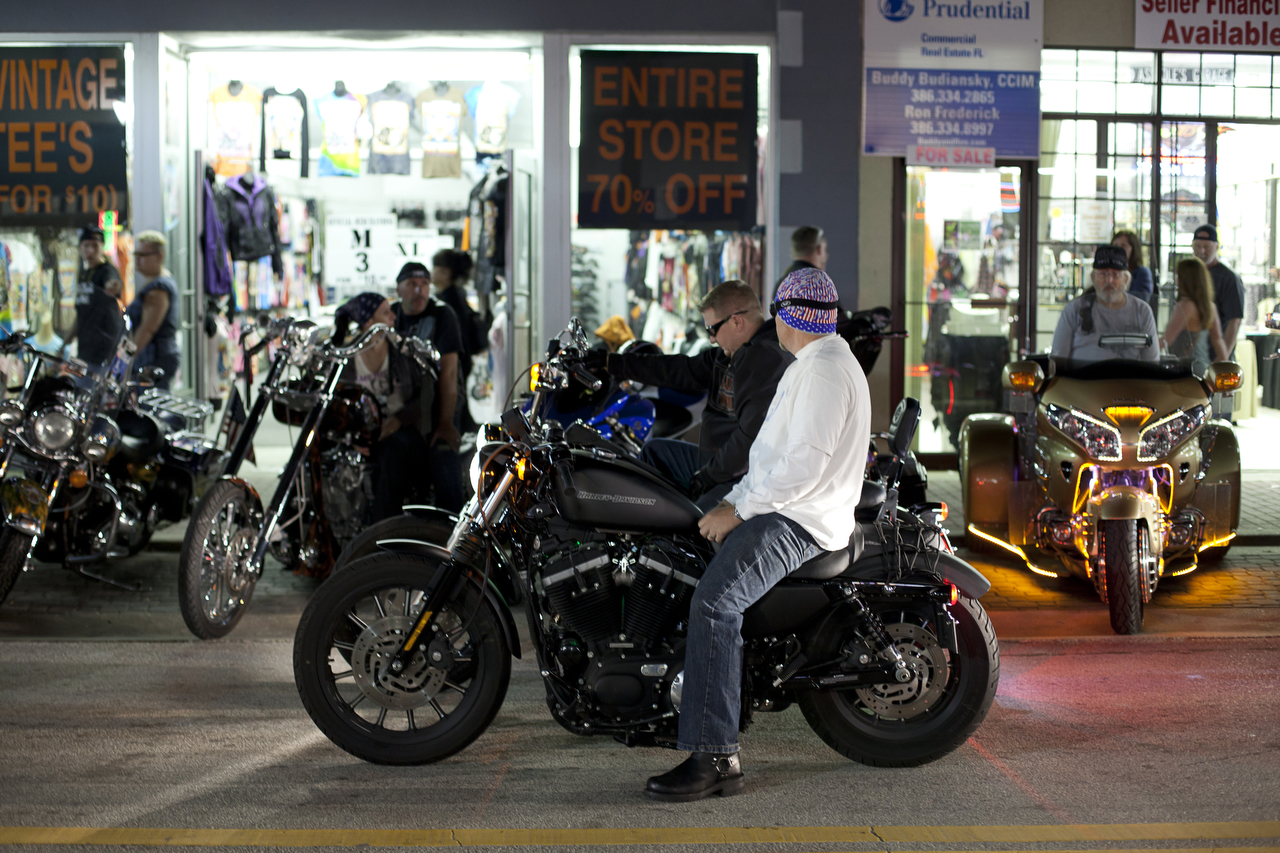The image depicts a nighttime scene with a group of at least six motorcycles, four of which have riders on them—a mix of men and women. The focal point is a man in the foreground wearing a white long-sleeve shirt, blue jeans, black boots, a purple hat, and goggles. This group of bikers, mostly white men, is parked outside a brightly lit store, which is adorned with various sale signs, including "Entire Store 70% Off" and "Vintage Tees for $10." The store's interior is visible through the windows, showing people shopping and walking around. Adjacent to this store is another shop with its lights on and a Prudential sign, indicating its availability. The scene has a vibrant contrast suggesting it's nighttime, and the bikers appear to be waiting, possibly for others to exit the store.